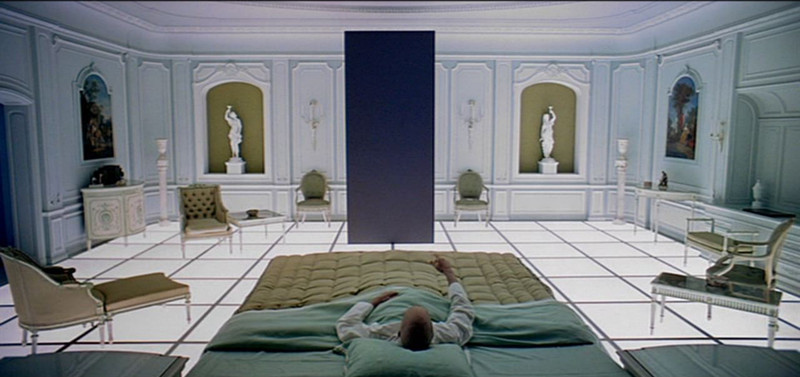The image depicts a vast, intricate room with a white tile floor and white walls, resembling a Victorian-style museum or mansion. The luxurious space contains an array of Victorian furniture, including several one-person seats, a bench, and a daybed-like seat. Statues are displayed in alcoves, and paintings adorn the walls on both the left and right sides. The color palette of the image includes pale baby blue, army green, and sea foam green.

In the center of the room stands a prominent blue triangle, and a large black rectangle or screen is also noticeable within the space. At the bottom center of the image, a man lies in an Asian-styled, queen- or king-sized bed with no mattress, covered by green bedding. The man, wearing a light blue top, is viewed from above his head, facing the vertical black screen. Flanking the bed on both sides are two wooden dressers or small tables. Despite its vast and open layout, the room feels intimate yet grandiose, blending elements of a sophisticated home with the ambiance of an art gallery.